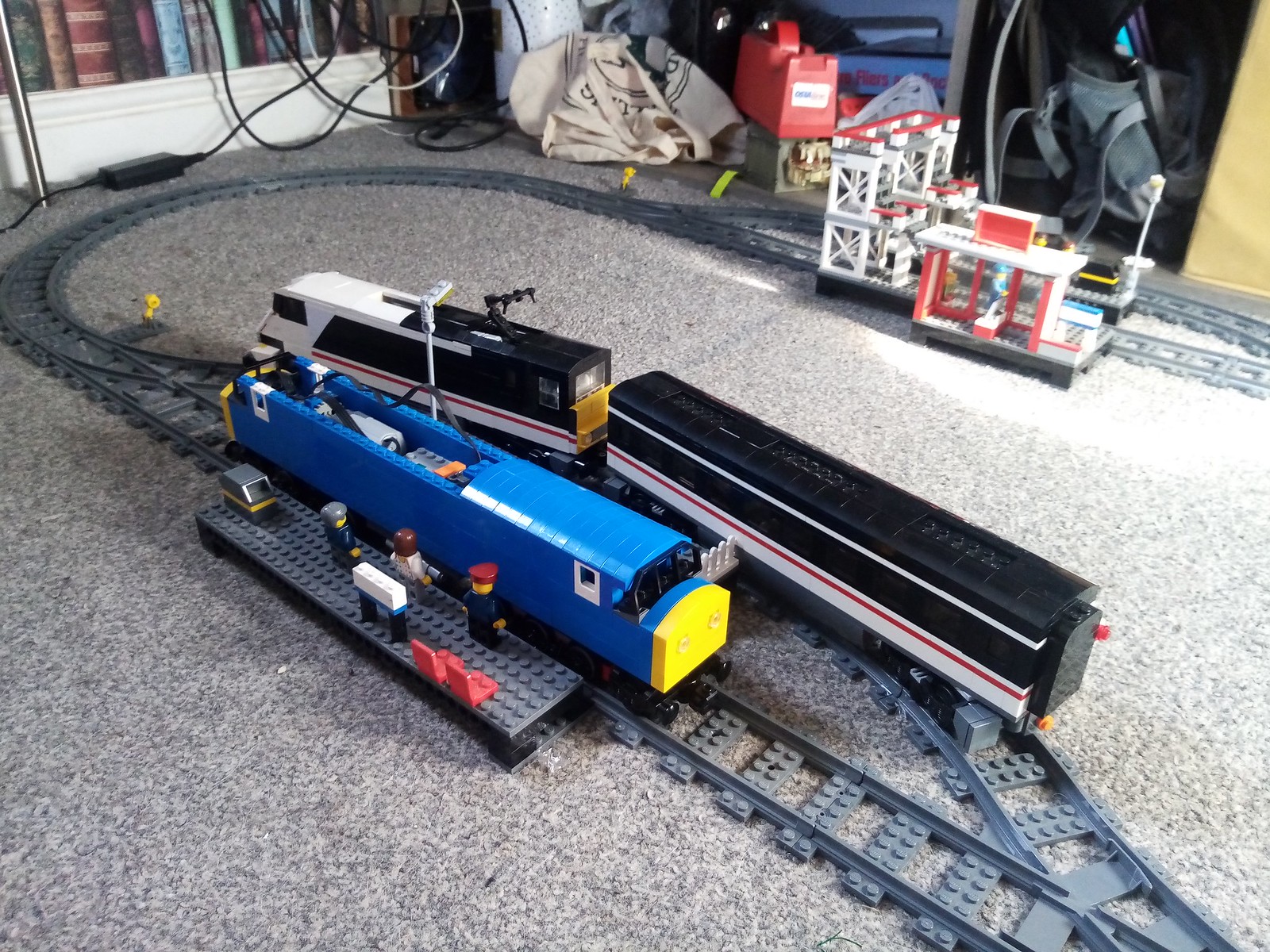The image depicts a detailed toy train set arranged on a gray Berber carpet, set up in what appears to be a room inside a house. The train set comprises a large oval track that extends beyond the right edge of the frame. On the track, there is a bright blue plastic train car with a yellow front, drawing immediate attention. Following this car are two additional train cars; one is white and black, and the other is black with white and red stripes, both of which have large windows along their sides. In the scene, small wooden figurines populate a waiting area platform with red seats and an awning featuring a sign, where a little conductor figurine with a red hat stands alongside another figure with gray hair and a blue shirt.

The environment around the train set includes a white bookcase filled with books located in the top left corner of the image. Scattered near the tracks are various items, such as a backpack, a jug that might hold gasoline, and other tote bags. A potential closet is hinted at in the background to the right, possibly housing a golf or tote bag. The carpet underneath is a mix of gray and black, resembling a peppered texture, complementing the vibrant colors of the train set and its accessories.